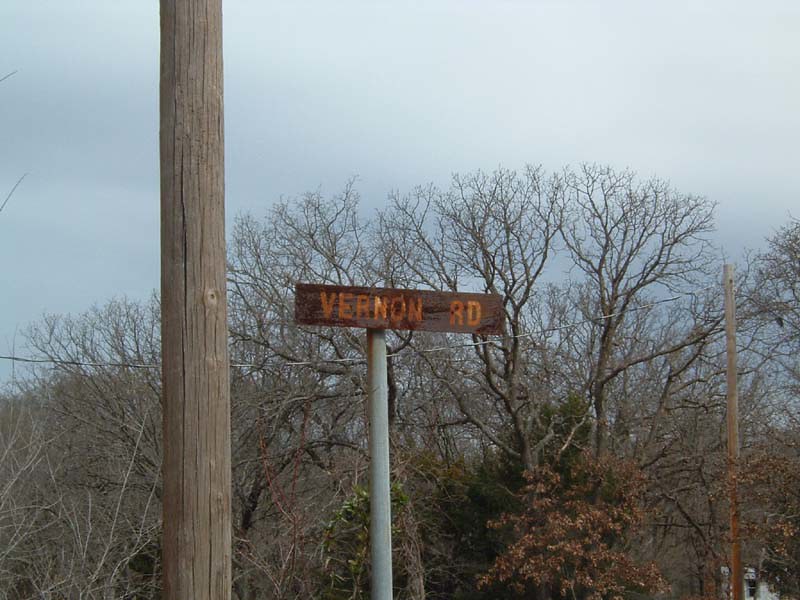In this image, we see a weathered street sign for "Vernon Road," characterized by its orange lettering against a brown background. The sign appears temporary and mismatched with the thick pole it is attached to, giving an impression of a makeshift setup. The street sign is positioned beside a very tall telephone pole, whose top is out of the frame, with another telephone pole visible to its right. Leafless tree tops in the background suggest a winter setting, echoed by the presence of a smaller tree with brown leaves. The image also captures the overhead wires strung between the telephone poles, under the backdrop of a cloudy sky.